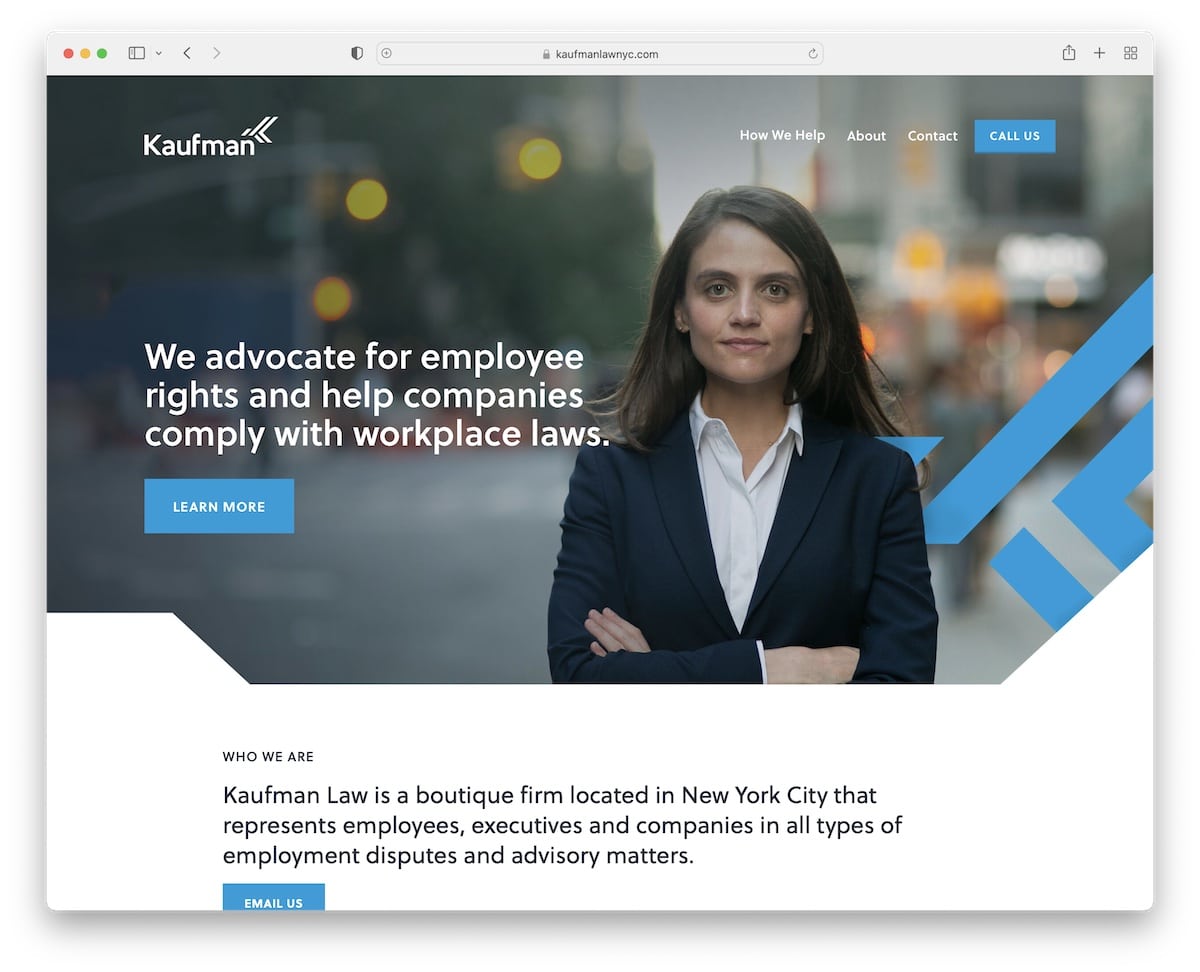This is a detailed capture of a website's interface. At the top, there is a gray navigation bar featuring three circles in red, gold, and green sequentially. It also includes various icons such as a tablet symbol, a down arrow, a back arrow, a forward arrow, a shield symbol, a plus sign within a circle, a padlock icon, and a web address field. To the right, there's a refresh button, depicted as a square with an arrow, and a plus sign alongside four small squares.

Below the navigation bar, the name "Kauffman" is prominently displayed in white text, accompanied by a small arrow icon. Adjacent to this are navigational links in white that read "How We Help," "About," and "Contact," while a "Call Us" button appears in blue and white.

In the main section of the webpage, there is an image of a woman. She has brown hair and is dressed professionally in a white dress shirt and a navy blazer, with her arms folded. Overlaid on the image, a white text states, "We advocate for employee rights and help companies comply with workplace laws." Below this message, there's a "Learn More" button in blue and white. In the background, slightly blurred, there is a blue checkmark near her shoulder, stoplights with a yellow hue, and some indistinct buildings.

Further down, black text announces, "Who We Are," followed by a description: "Kauffman Law is a boutique firm located in New York City that represents employees, executives, and companies in all types of employment disputes and advisory matters." A blue and white box with the text "Email Us" is situated beneath this description.

The overall website design features bold and easy-to-read fonts, ensuring user-friendly navigation and readability. The image captures all relevant and visually interesting elements of the webpage.